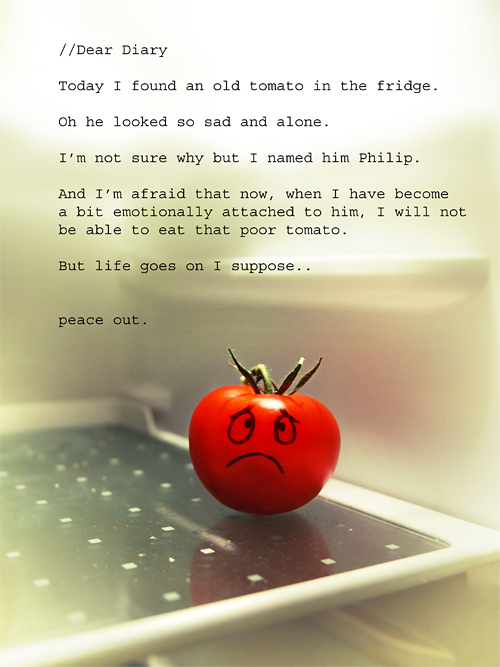In this image, we see a tomato sitting alone on an empty, slightly dirty refrigerator shelf with a clear plastic top. The refrigerator's off-white sidewall frames the space. The tomato, drawn with a sad face using a sharpie, has two eyes with pupils positioned towards the upper edges, giving it a forlorn expression, accentuated by downturned lines for the mouth and furrowed eyebrows. The tomato still has its green leaf stems on top, adding to its character. Above this scene, a letter is written: "// Dear Diary, Today I found an old tomato in the fridge. Oh, he looked so sad and alone. I'm not sure why, but I named him Philip, and I'm afraid that now, when I have become a bit emotionally attached to him, I will not be able to eat that poor tomato. But life goes on, I suppose. Peace out." The overall composition brings emphasis to the bright red tomato, making it the focal point against the faded background.